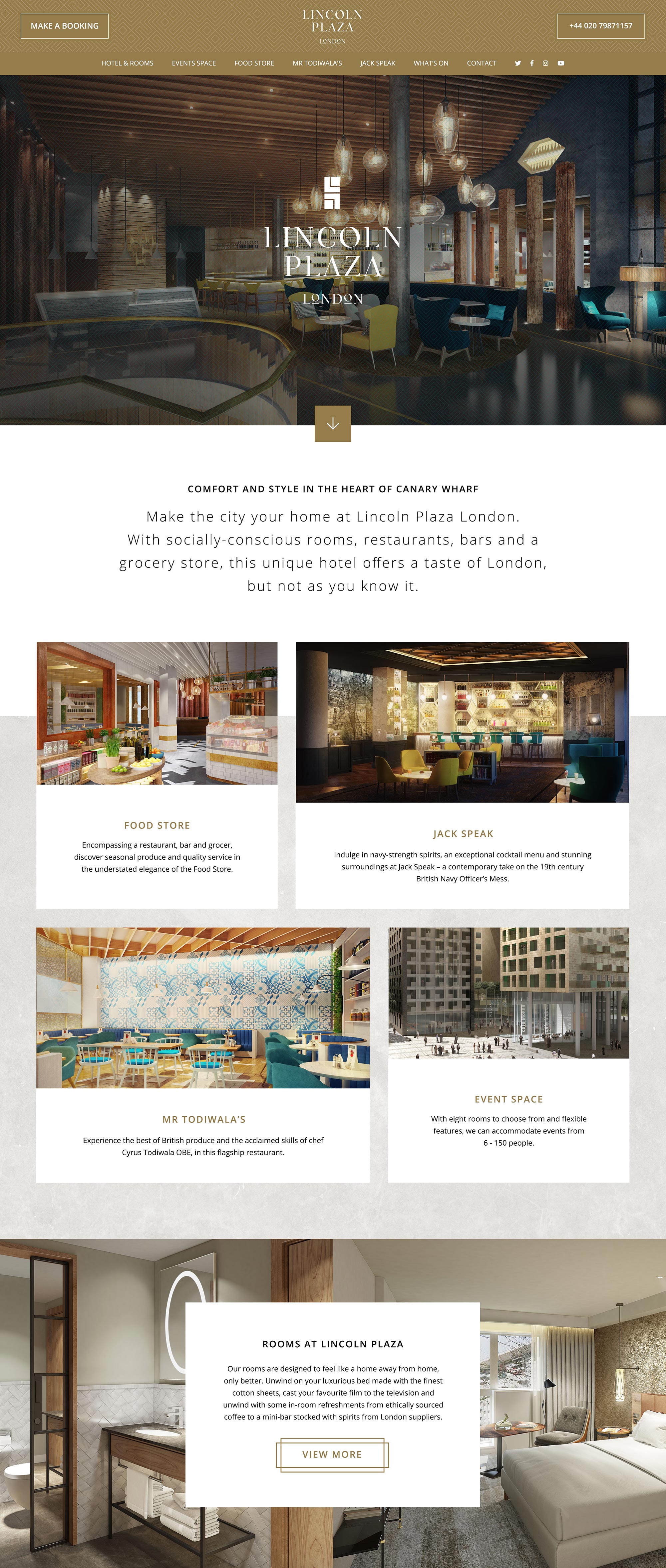This is a cropped screenshot of the Lincoln Plaza Hotel home page displayed in mobile landscape format, presenting a comprehensive view of the entire page in a single frame. The layout is designed to fit within a narrow screen, emphasizing its suitability for mobile viewing. 

At the top of the page, a photograph showcases a stylish and modern hotel interior with a warm and inviting ambiance. Centered over this image is a white text overlay that reads "Lincoln Plaza," prominently marking the hotel's name.

Beneath the main header image, a succinct description of the hotel appears in black font, providing an introduction to potential guests. Following this text section, there are four smaller thumbnails arranged over a gray square background. Each thumbnail is accompanied by a white box below it, containing brief descriptions of the hotel's various amenities.

Towards the bottom of the page, two horizontally aligned images offer an overview of the hotel's facilities: one displaying a detailed view of a bathroom, and the other showcasing an angled shot of a guest room. Centrally positioned over these images is a white pop-up box featuring a distinct "Book Now" button at the bottom, encouraging immediate reservations.

The design and layout effectively combine visually appealing elements and concise information, making it easy for users to navigate and engage with the hotel's offerings.